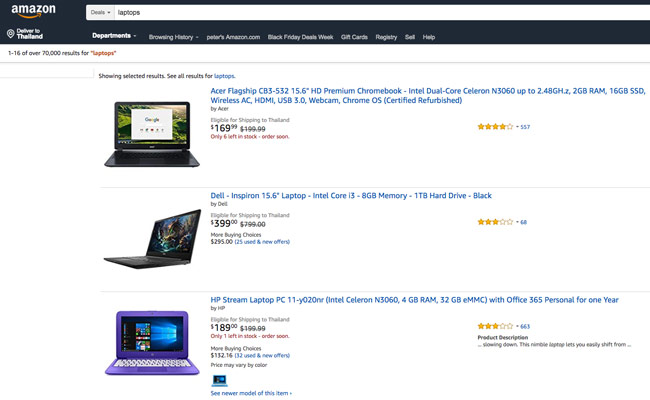The image depicts an Amazon webpage where a user has searched for laptops. At the top of the page, the search bar is white with a navy blue background. "Amazon" is prominently displayed in white text with a yellow arrow pointing upward. Just below the search bar is a navigation bar showing the search results for laptops.

Three laptop listings are visible:

1. The first listing is for an Acer Flagship 683532 computer. The title is clickable and written in blue. It shows a price, stock availability, and four-star reviews.
2. The second listing is for a Dell Inspiron 15.6 laptop, featuring an Intel Core processor. This black laptop has three stars and is priced at $399.
3. The third listing is for an HP Stream PC priced at $189. The description is written in black, with additional text in red. This purple laptop also has three stars and 663 reviews.

The detailed search results provide essential information such as product names, prices, customer ratings, and stock availability for the user to make an informed purchasing decision.